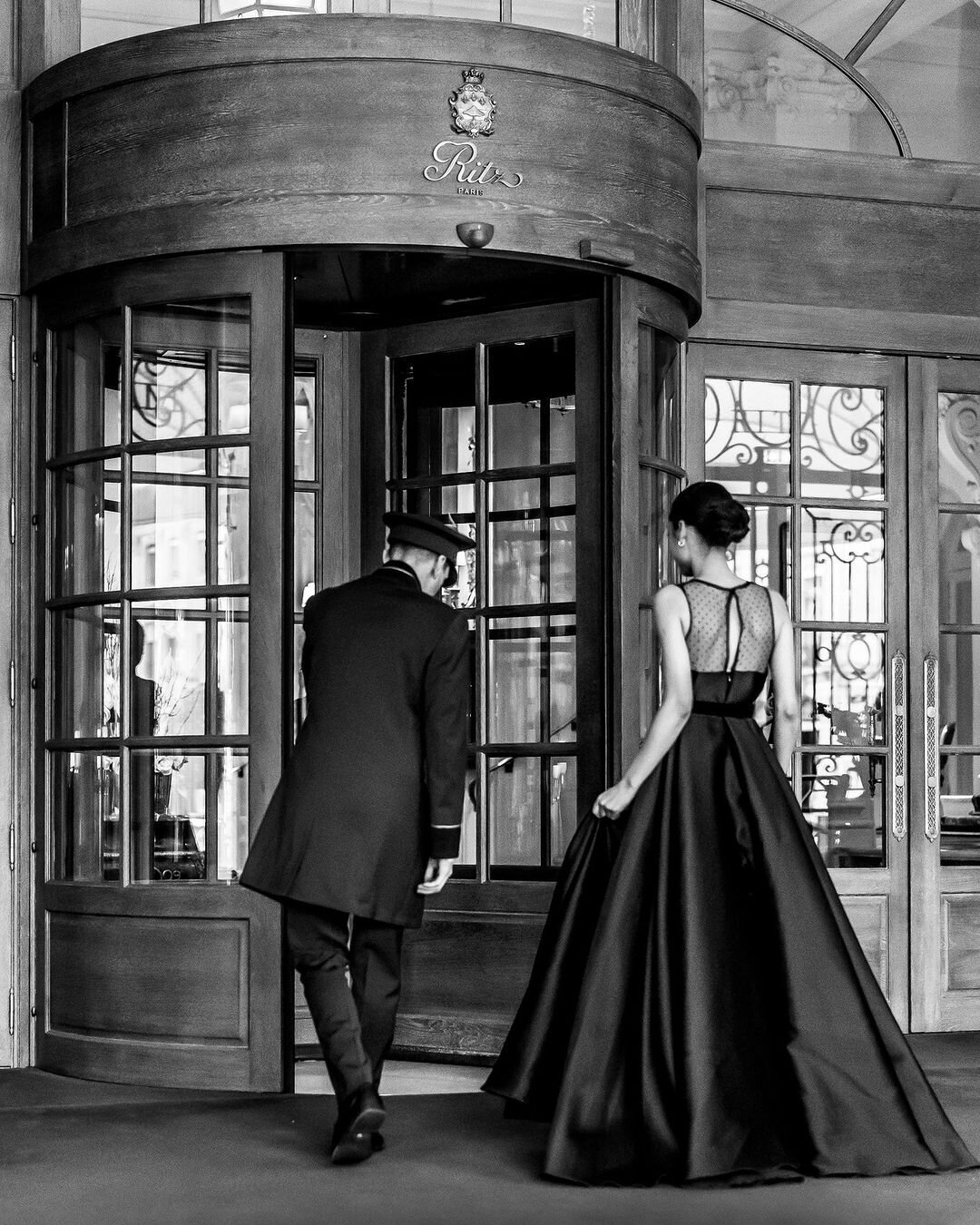This black-and-white photograph, designed to emulate an old-fashioned style, captures a moment outside the entrance of the Ritz Hotel in Paris. In portrait orientation, the image features a woman in her thirties, seen from behind, as she steps into the hotel's revolving door. She is adorned in a long black satin ball gown with a sheer, backless center and an a-line skirt that flows to the floor. Her dark hair is elegantly styled in a bun at the nape of her neck.

To her left stands a bellhop, dressed in dark attire with a long jacket and a hat, assisting her by holding the revolving door. His head is slightly bowed as he performs this task. The revolving door itself is a cylindrical booth with curved wood at the top and bottom, and glass panels. Above the door, a sign reads "Ritz Paris" in gold script with a crown-shaped coat of arms above it.

On the right side of the image, double doors with large glass windows and handles at the center are visible. The photograph also captures the reflection of an ornate iron gate in these windows. The overall composition of the image emphasizes the grandeur and elegance of the hotel's entrance, enhanced by the timeless black-and-white aesthetic.